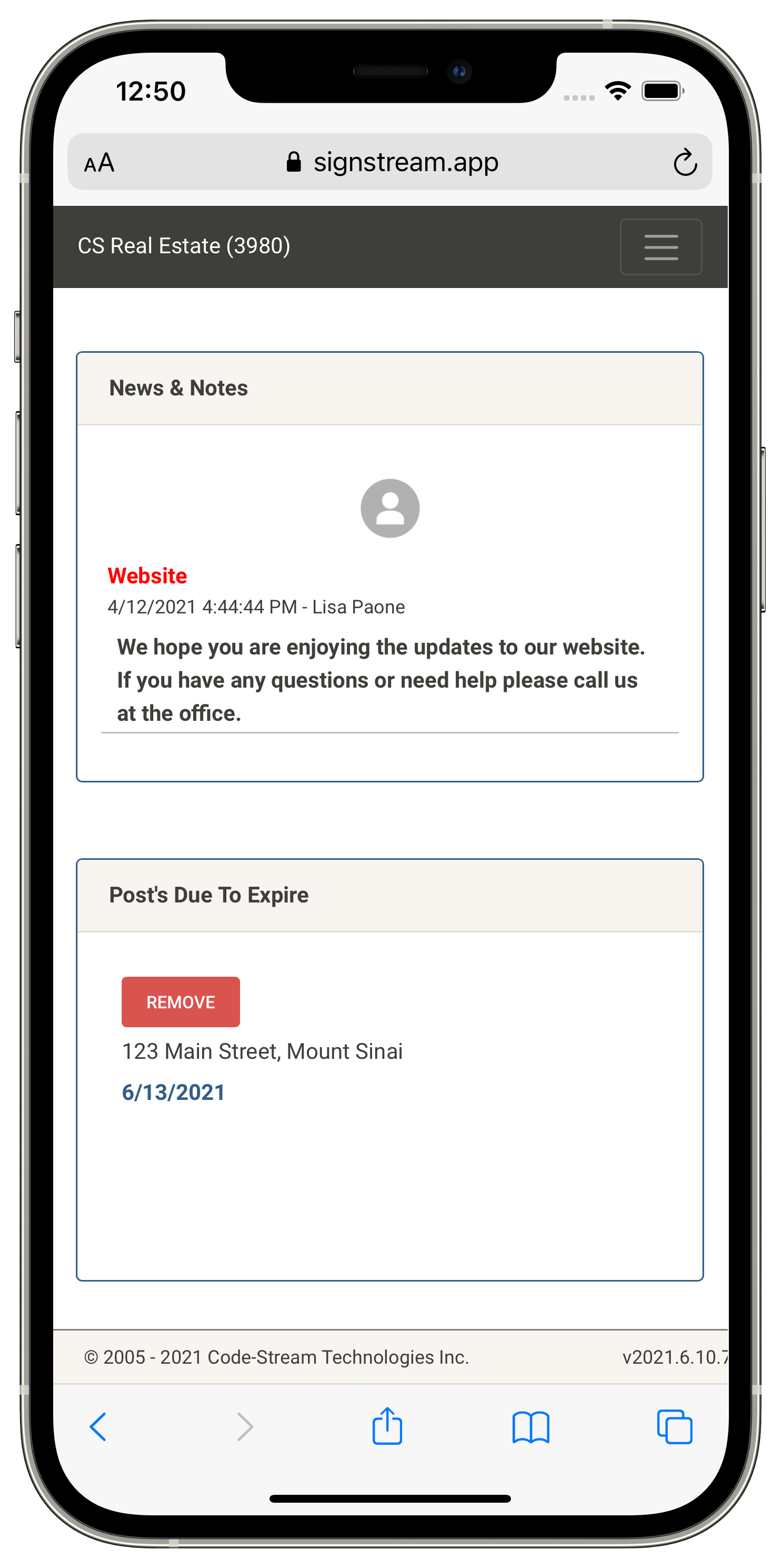This is a detailed description of a webpage displayed on a white cell phone with a full battery and a strong connection, captured at 12:50. The webpage belongs to SignStream.app, evident from the address in the search bar at the top, where there is also an "AA" icon on the left and a circular arrow icon on the right. Below these, the header reads "CS Real Estate" in black text on a black strip, next to an icon featuring three horizontal lines.

The screen features a gold-tinted bar labeled "News and Notes." Within this bar is an icon of a person and red text saying, "We hope you're enjoying the updates to our website. If you have any questions or need help, please call us at the office."

Below this announcement lies another section with a blue-dotted border titled "Posts Due to Expire." Inside this box is a red button labeled "Remove," alongside information about a specific post: "123 Main Street, Mount Sinai, 6/13/2021."

The bottom of the phone displays the standard icons seen on most cell phones, completing the familiar user interface.